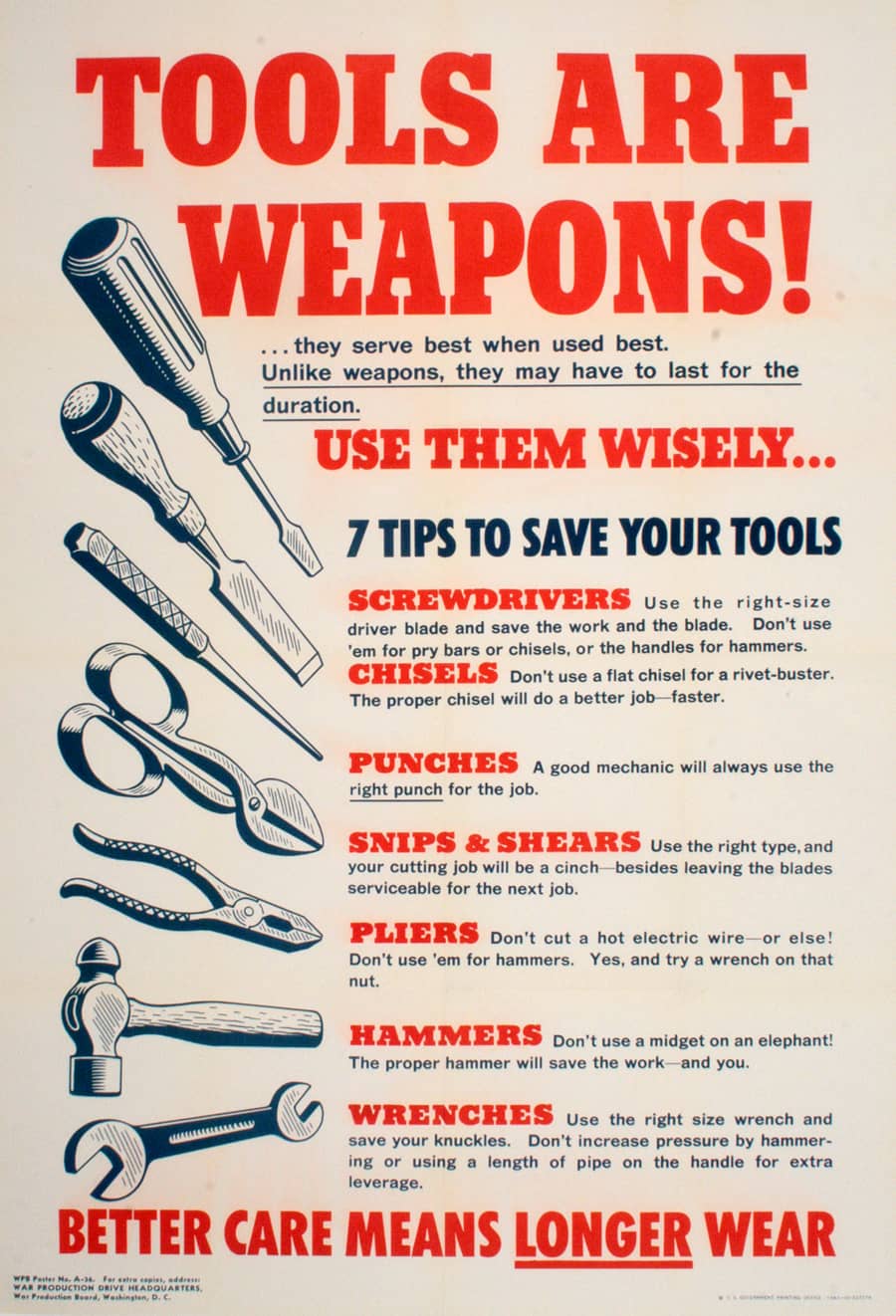The poster features a detailed and colorful layout aimed at promoting proper tool care. At the top, bold red capital letters announce, "TOOLS ARE WEAPONS!" Below this, blue underlined text states, "They serve best when used best. Unlike weapons, they may have to last for the duration."

Down the left side of the poster, illustrations of various tools are displayed, including different sizes of chisels, a pair of pliers, a hammer, a wrench, and some scissors. The right side continues with instructional text in alternating red and blue letters. 

The message "Use them wisely" appears in red, introducing seven tips to save your tools. Each tip highlights a different tool with corresponding guidelines:

1. **Screwdrivers:** Use the right size driver blade to protect the work and the blade. Avoid using them as pry bars, chisels, or hammers.
2. **Chisels:** Don't use a flat chisel for a rivet buster; the appropriate chisel will do the job faster and better.
3. **Punches:** A good mechanic uses the right punch for each task.
4. **Snips and Shears:** Use the correct type to make cutting easier and preserve the blade for future use.
5. **Pliers:** Do not cut hot electric wires with pliers, avoid using them as hammers, and choose a wrench for turning nuts.
6. **Hammers:** Select the proper hammer for each job to avoid overexertion and damage.
7. **Wrenches:** Use the correct size wrench to save your knuckles and avoid using pipes for added leverage, which can cause damage.

At the bottom of the poster, the phrase, "Better care means longer wear," emphasizes the theme of tool preservation.